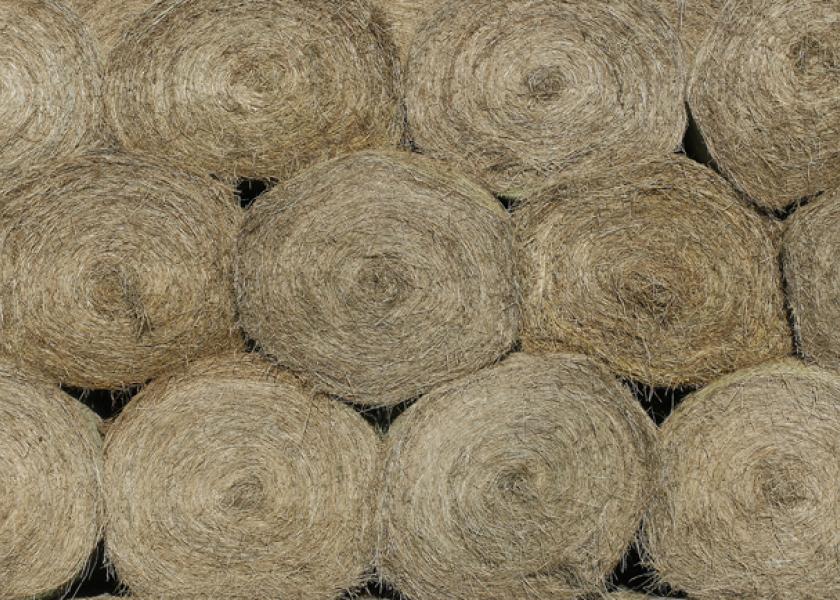This image displays a top-down view, possibly taken by a drone, of twelve large, beige bales of hay densely packed and stacked in three rows of four each, positioned on a dirt ground. The cylindrical bales exhibit a spiral texture, reminiscent of cinnamon rolls, with darker centers and lighter, earthy hues towards the edges. The rough texture of the hay rolls indicates their likely use for feeding animals or planting seeds. Gaps between the bales reveal small patches of earth, adding to the rustic farm setting. The overall composition is simplistic yet striking, highlighting the natural, unrefined beauty of the hay bales.